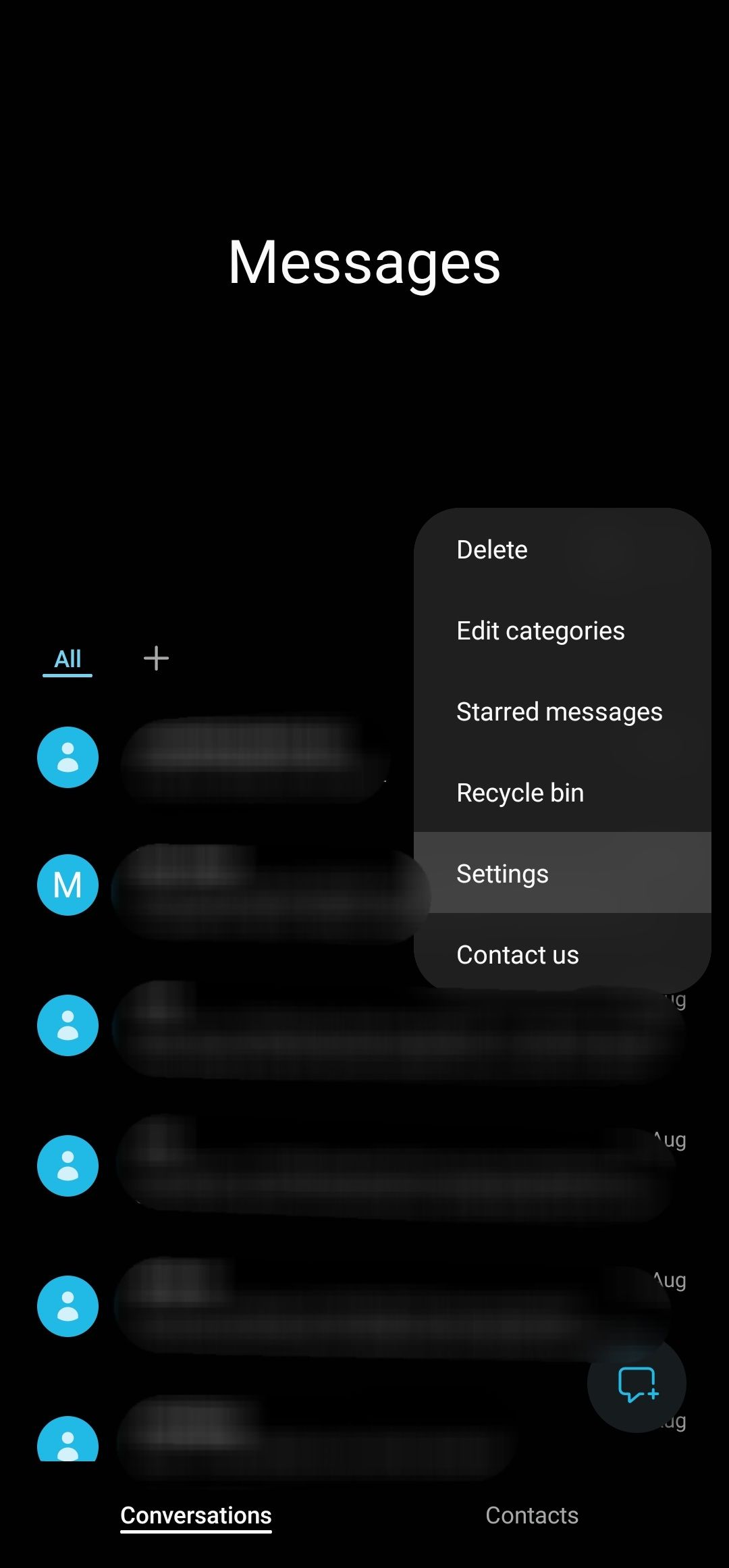A dark mode interface displays a messaging app titled "Messages" at the top. The background is black, making the white text and minimalistic graphics stand out. The screen shows multiple conversations between individuals, represented by generic profile icons. The identity of the senders and recipients remains anonymous, denoted only by initials such as "M," with all message content censored and blurred out. Visible timestamps suggest messages were exchanged in August, indicated by an "AUG" label to the side. 

An additional settings menu is open following a long-click on a message, offering options such as delete, edit categories, share, star messages, recycle bin settings, and contact us. At the bottom of the interface, there are two tabs: "Conversations" (currently active) and "Contacts." The "Conversations" tab is highlighted with a blue icon portraying a simplistic, generic silhouette of a man's head and upper torso.